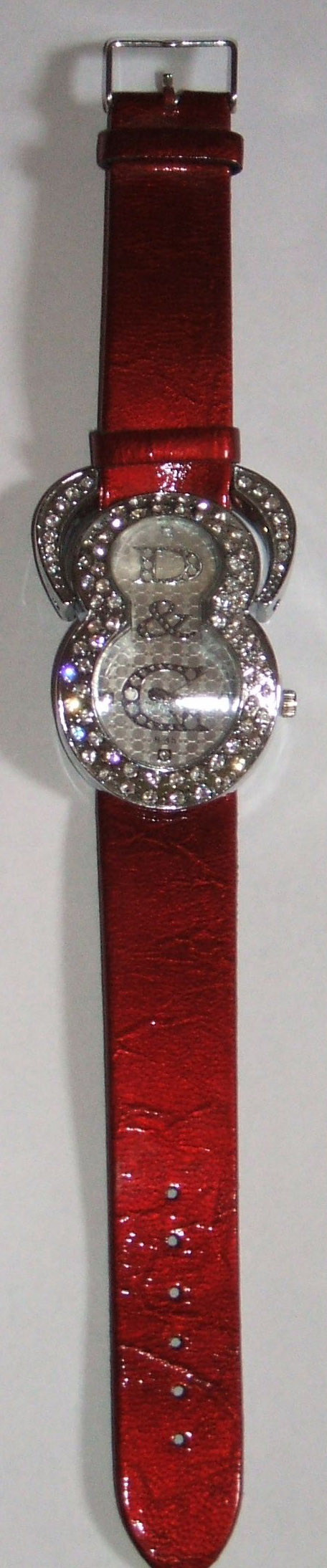This image showcases an elegant, designer watch positioned vertically against a stark white background, occupying the entire frame. The watch features a vibrant red leather band that lends a striking contrast to the minimalist setting. At the top of the watch, a sleek silver buckle gleams, hinting at its high-quality craftsmanship. 

Cleverly designed to catch the eye, the watch face is uniquely shaped like the number 8, adorned with a dazzling border of rhinestones that add a touch of opulence. The dial boasts a shimmering silver hue, complemented by rhinestone initials "D" and "G" at the center, suggesting the watch is a product of the renowned Dolce & Gabbana brand. Rhinestones not only frame the watch face but also embellish its interior, creating a seamless blend of luxury and style. The subtle shadow cast beneath emphasizes the watch’s three-dimensionality, making it appear even more realistic and tangible.